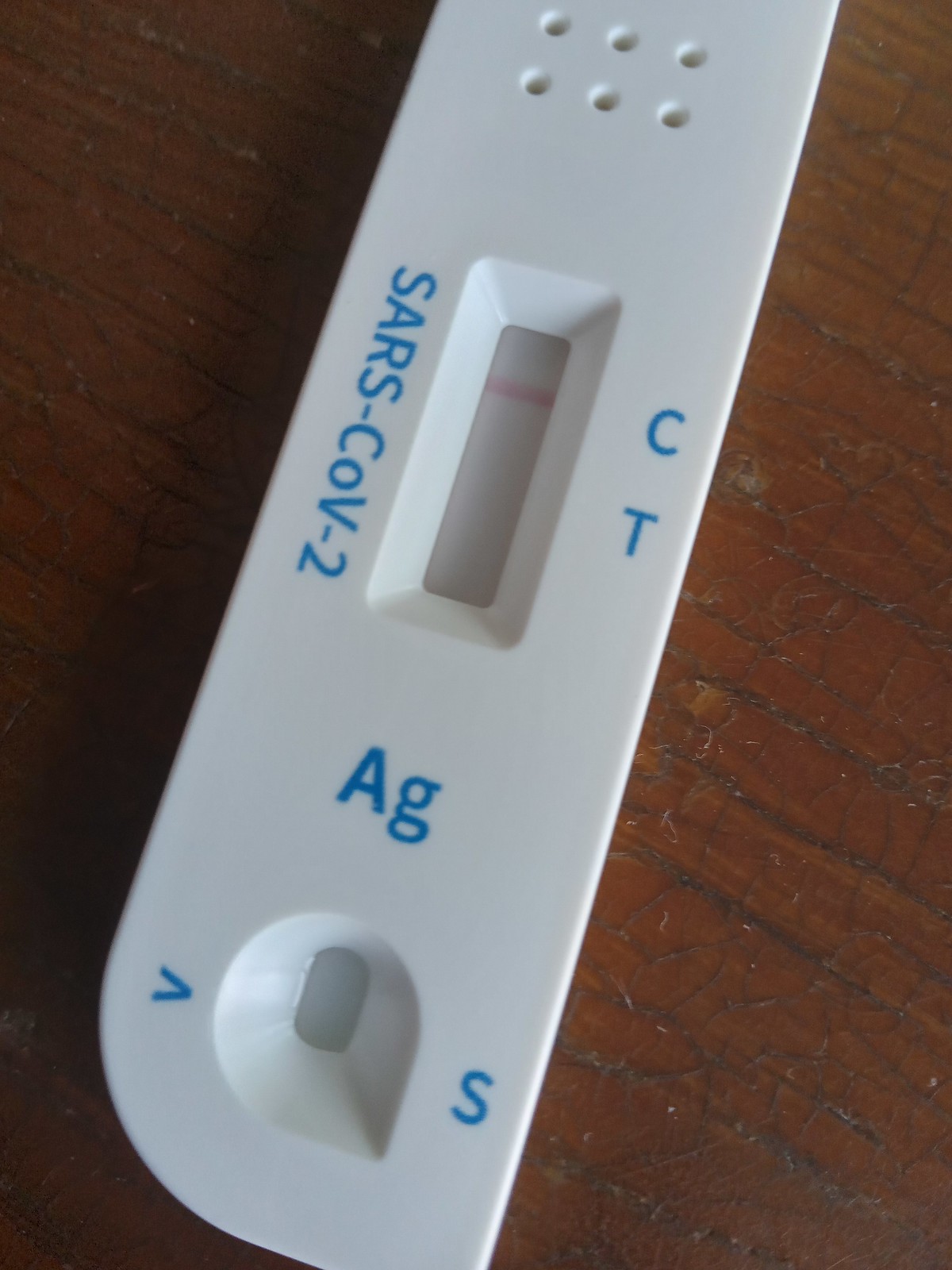A close-up image showcases a COVID-19 rapid test resembling a plastic pregnancy test device. The test features a rectangular, white plastic body with six small circular openings along the top, possibly designed for ventilation. On the left side, the label reads "SARS-CoV-2" in blue print, while the right side displays a "C" with a pink line next to it and a "T" with no line, which indicates the test result. In the lower central section, the letters "AG" are prominently printed in blue. Below this, there's a funnel-like receptacle, likely where the sample is deposited. This area is flanked by the letters "V" on the left and "S" on the right. The device rests on a wooden surface, identifiable by the visible wood grain of what appears to be a countertop or table.